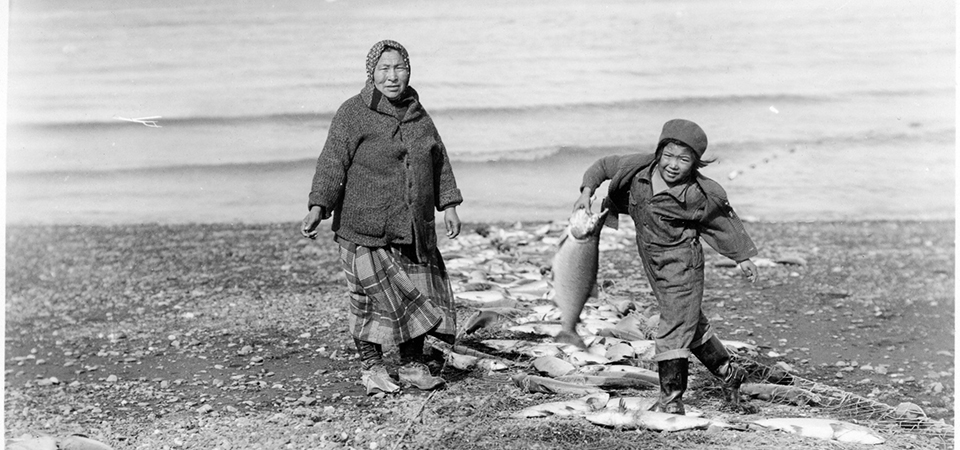This horizontally aligned, older black-and-white photograph captures a poignant moment by the shoreline with choppy waves in the background. The beach in the foreground appears dark and rocky, sparingly scattered with small stones. In the center of the image stand two figures. An older woman is dressed warmly in a dark, woolen coat, a plaid skirt, and tightly laced-up boots, with a headscarf or head wrap. Her gaze meets the camera directly. To her right, a young boy, approximately ten years old, joyfully holds a large fish by its mouth. He seems to be struggling to walk sideways, possibly due to his heavy, woolen one-piece suit and sturdy boots designed for wet environments. Numerous dead fish lie strewn across the ground between the two, leading from the water's edge to the photograph's bottom. The boy’s expression is one of pride and excitement as he lifts the fish, and both figures are framed by the natural, albeit harsh, coastal scenery.